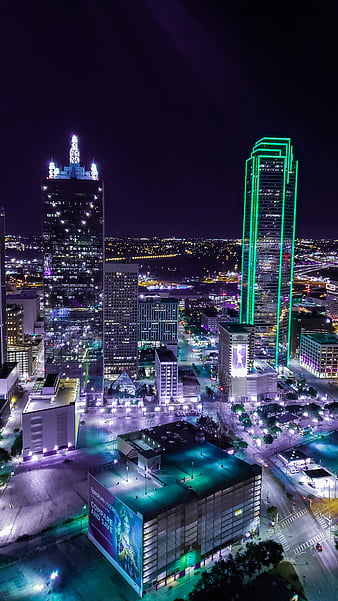This vibrant nighttime photograph captures an aerial view of a bustling city skyline with numerous skyscrapers illuminated against the dark sky. Dominating the foreground is a rectangular building featuring an advertisement with a woman on the right side and the text "compare and save" on the left. Adjacent to this building, on the left, stands a striking black glass skyscraper adorned with illuminated crosses, crowned by a series of blue and white lights at its pinnacle. To the far right, another prominent skyscraper is outlined with green neon lighting, adding a distinct glow to the scene. The lower part of the image reveals city streets awash in hues of purple, blue, white, and green neon lights, highlighting the city's vibrant nightlife. The sky above is a void of any celestial bodies, emphasizing the urban environment's artificial illumination.